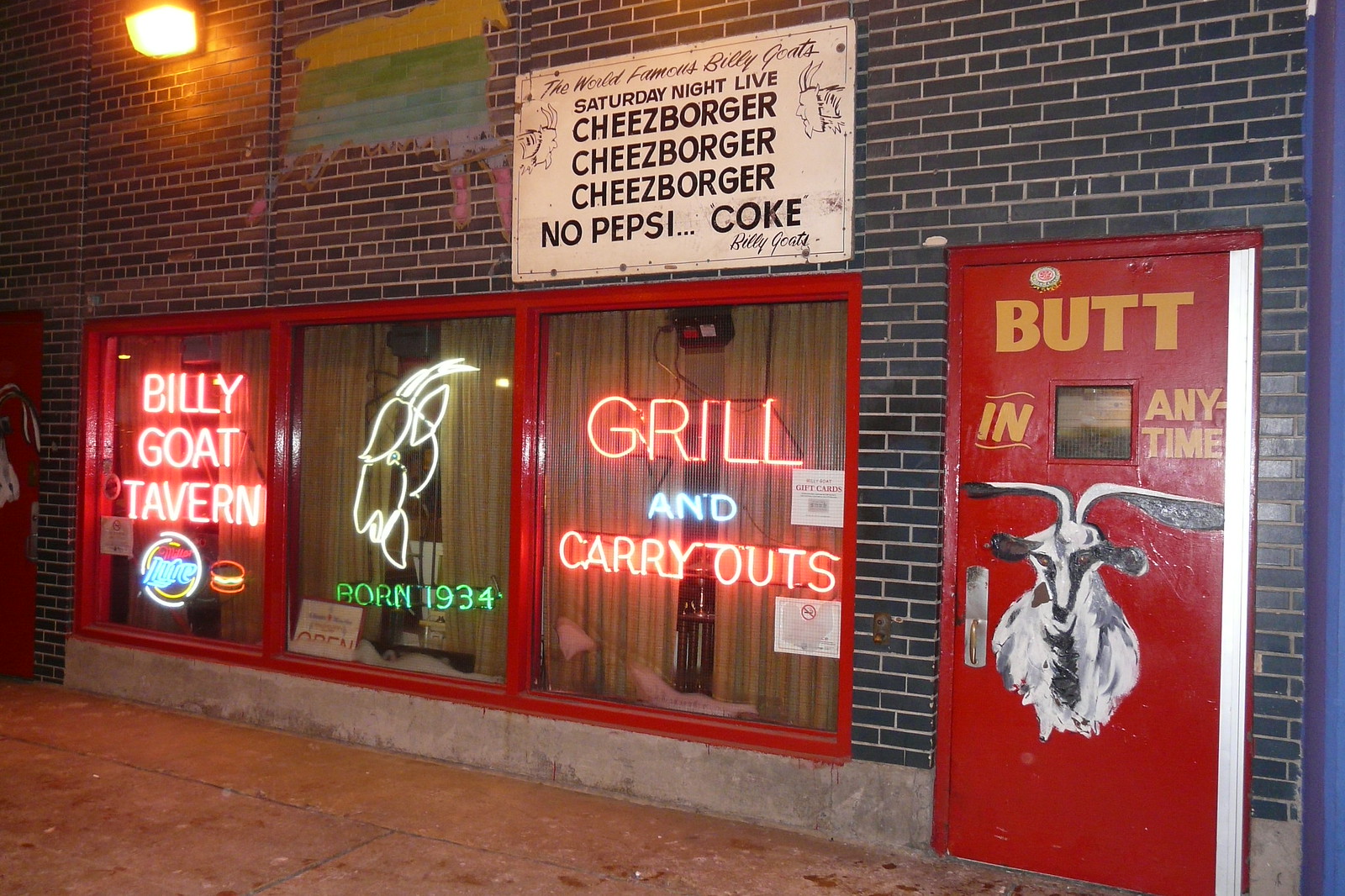This photograph depicts the vibrant exterior of the Billy Goat Tavern, a bar that encapsulates a rich sense of history and character. The front facade of the establishment showcases a striking combination of red, yellow, and blue hues. Made to resemble blue brick, the building’s wall exudes an eclectic charm. Three large windows trimmed in red dominate the scene.

The leftmost window features red fluorescent lettering that reads "Billy Goat Tavern," accompanied by the Miller Lite logo and a neon illustration of a cheeseburger. The center window displays the neon outline of a goat's head, glowing white, with "Born 1934" illuminated in green below, and a sign indicating the tavern is open. The rightmost window, marked with red and blue neon, spells out "Grill and Carryouts" and is adorned with several papers, likely health code notices, posted up. A yellow curtain hangs inside, adding a hint of warmth to the window layout.

To the right of these windows is the entrance—a bold red door featuring a white-painted image of a goat from the shoulders up. The door includes a small window near its top and is emblazoned with the phrase "BUTT IN ANYTIME" in yellow lettering, divided on either side of the small window. The establishment’s playful spirit is further emphasized by a sign on the brick wall that reads "Saturday Night Live cheeseburger, cheese 'C-H-E-E-Z', borgor 'B-O-R-G-E-R', repeated three times, no Pepsi, Coke, Billy Goat."

The lower part of the building is bordered by cement, and the street in the foreground further frames this lively and inviting entrance. This detailed and colorful facade invites patrons to step inside and experience the spirited atmosphere of the Billy Goat Tavern.